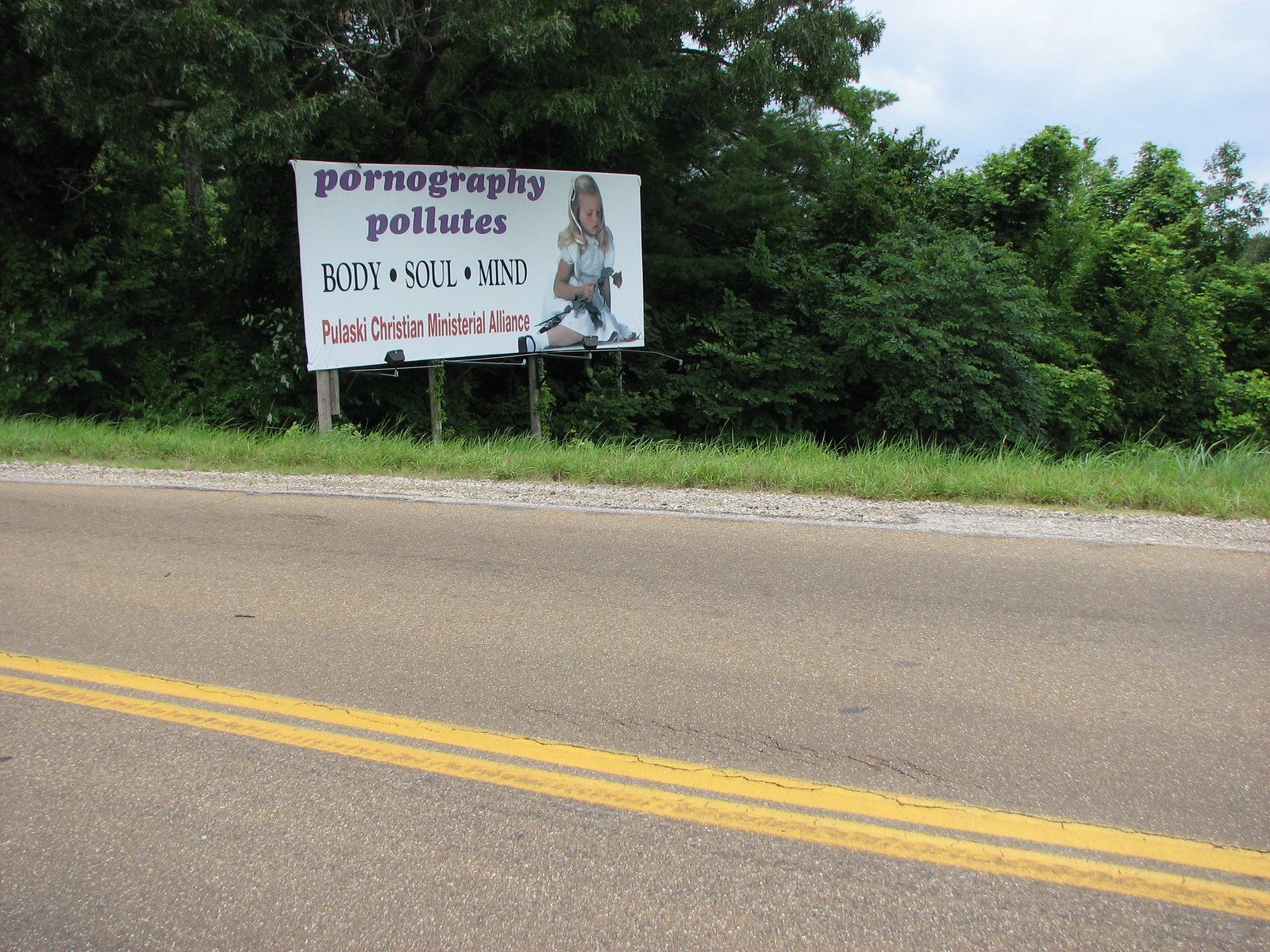The photograph captures a roadside scene prominently featuring a large, white-background billboard supported by wooden posts with ivy growing around them. The billboard displays a clear anti-pornography message in distinct, multi-colored text. At the top, the words "Pornography Pollutes" are written in purple. Below this, in black lettering with filled black circles between the words, it reads "Body • Soul • Mind." At the bottom, in red text, "Pulaski Christian Ministerial Alliance" is displayed. The billboard also includes an image of a young girl with blonde hair, light skin, wearing a white dress and white ribbons in her hair, holding a red-topped rose with a dark green stem. 

The billboard is situated on the right-hand side of a light gray road with double yellow lines running down the middle, indicating separate directions. Surrounding this road on the right is a line of dark green trees and bushes. There's a patch of light green grass in front of the billboard, flanked by a thin line of light gray and dark gray gravel. The sky above is cyan blue with scattered white clouds, suggesting a very sunny day. The perspective of the photograph implies it was taken from within a vehicle, possibly from the backseat on the driver's side.